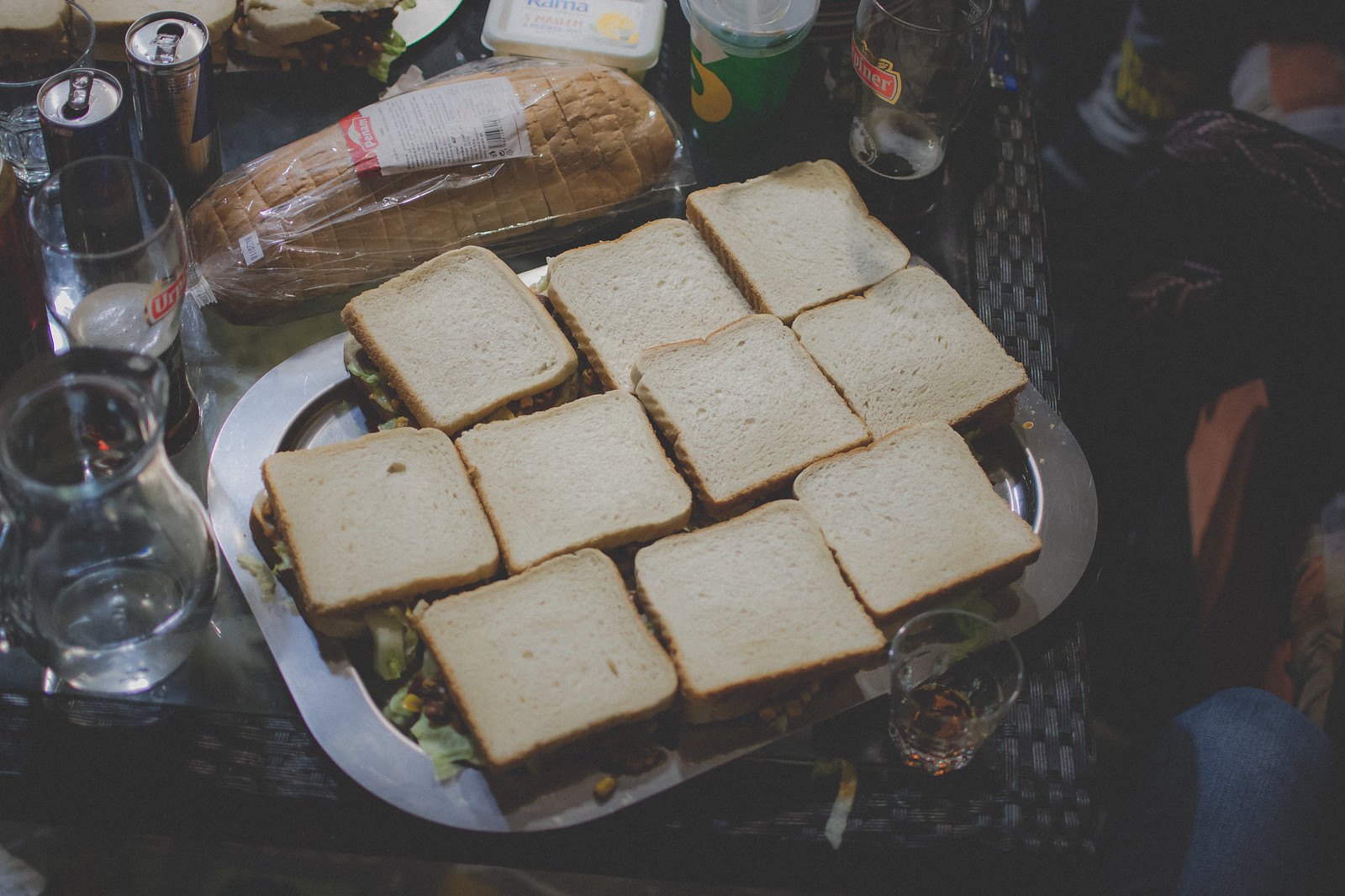The image shows a black or brown table adorned with a large silver tray at the center holding an array of neatly arranged sandwiches made with white bread, each stuffed with green lettuce. The sandwiches are organized into three rows, with three sandwiches at the top, four in the middle, and three at the bottom. Surrounding the tray, various items are placed on the table: on the bottom right, a glass filled with an orange drink, possibly soda or alcohol; to the back, a nearly empty beer glass; and a Subway cup positioned near what looks like a container of butter or cheese. Additionally, there is a loaf of bread in a bag on the left and a couple of Red Bull cans nearby. A couple of other beer glasses are also visible, suggesting a casually set eating and drinking environment. In the background, part of a dark pants leg can be seen, hinting at the presence of someone in the dimly lit setting.